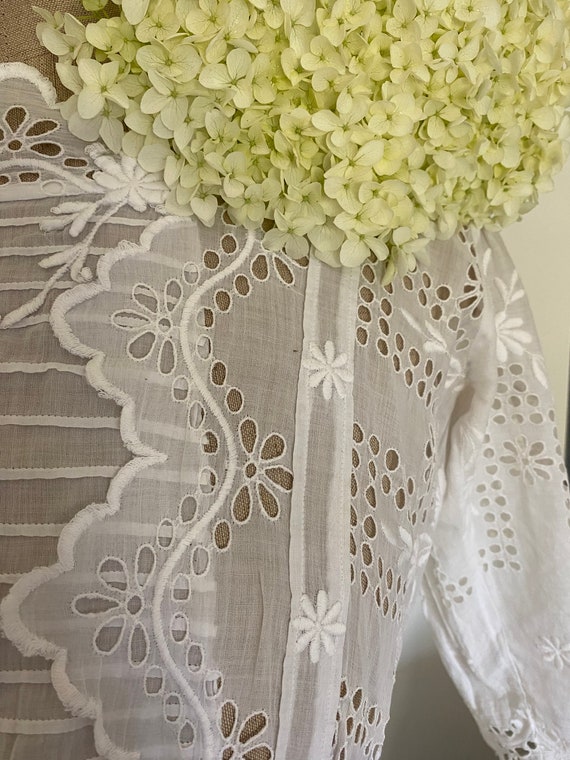The image depicts an intricate piece of bright white eyelet lace with floral embroidery, flower and circular cutouts. The lace is draped over what appears to be a mannequin or possibly a table, as interpretations vary. A creamy white hydrangea blossom, tinged with pale yellow against the stark white lace, is prominently positioned in the upper part of the image, creating a striking contrast. The background includes brown wood visible through the lace holes on the upper left, suggesting either a wooden table or part of a mannequin structure. A sleeve extends to the right, adding to the impression that the lace might be part of a garment. The overall background and setting offer a blend of beige, highlighting the complexity and elegance of the lacy textile and the delicate hydrangea bloom.